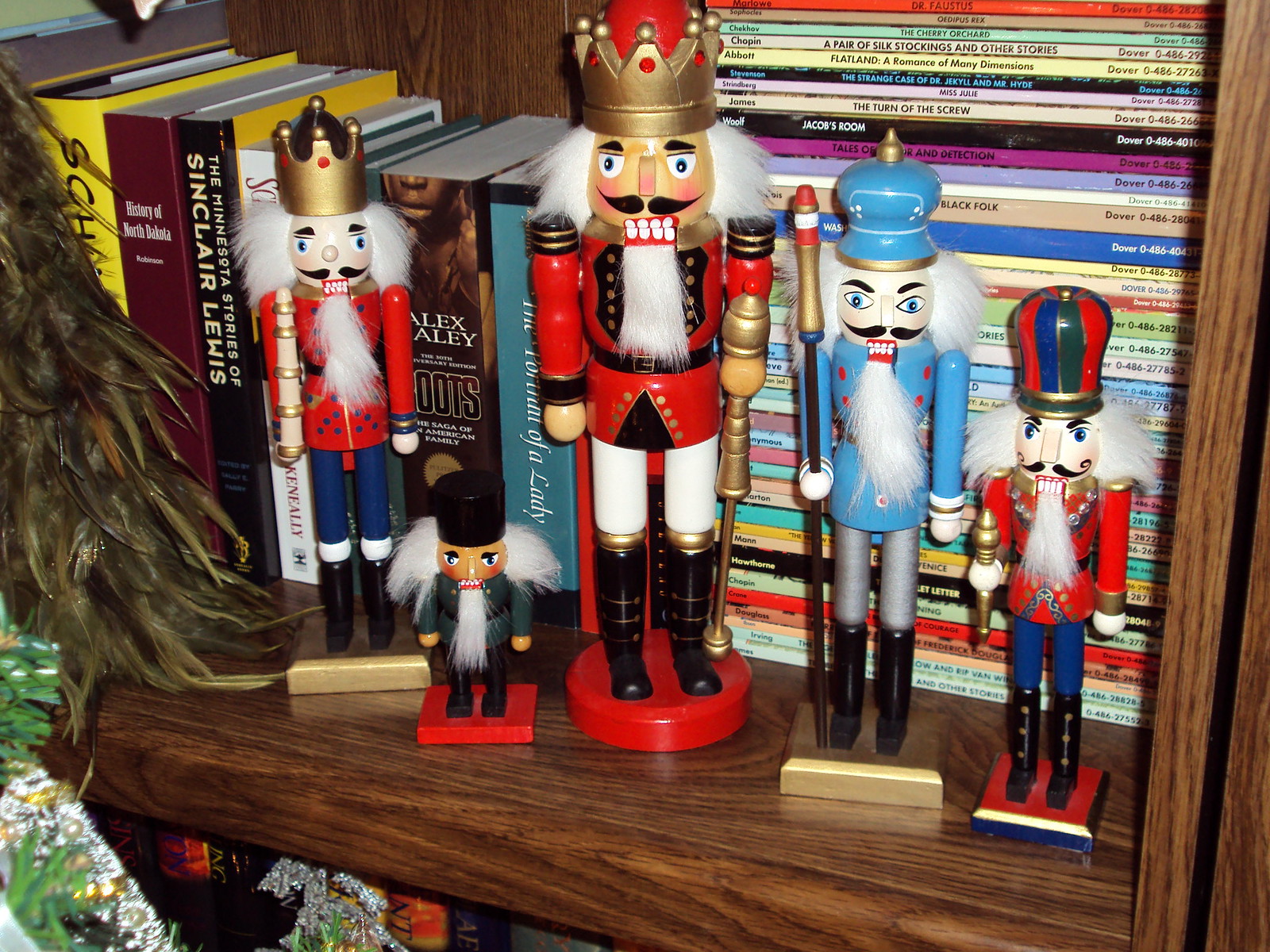This image captures a festive scene set against a bookshelf partially obscured by the branches of a Christmas tree on the left. The focus is a single shelf displaying a collection of five detailed nutcrackers, surrounded by neatly arranged books. The books are positioned both vertically and horizontally, with titles such as "Roots" and "The Turn of the Screw" visible on the spines.

The nutcrackers vary in size and attire, each with distinctive features:

1. The tallest nutcracker stands prominently in the middle. It has a red base, black boots with gold trim, white pants, and a white jacket. Its white beard and hair, black mustache and eyebrows, and a crown adorned with red jewels and gold circles make it stand out.
  
2. To the left of this tall nutcracker is a very small nutcracker, reaching about halfway up the tall one's height. It features a red square base, a black hat, a long white beard, white hair, a gray jacket, black pants, and black boots.

3. The leftmost nutcracker is of medium height, dressed in a red jacket, blue pants, and black boots with white cuffs. It stands on a gold base and sports a gold crown with red dots, a black beard, white hair, black eyebrows, and a long white beard.

4. To the right of the tallest nutcracker is a nutcracker dressed in an aqua blue outfit, matching hat with a gold point, silver pants, black boots, and a gray jacket. It holds a long sword in its right hand and stands on a gold square base.

5. The rightmost nutcracker, similar in height to the medium one on the left, shows a vibrant red uniform with gold trimmings, blue pants, black boots with bronze dots, and a multicolored crown resembling a hat. This nutcracker also features white hair and a white beard.

Books are stacked vertically on the far left while thinner books lie horizontally to the right, immediately behind the nutcrackers. Overall, the scene gives a warm and festive feel, emphasizing the holiday atmosphere.